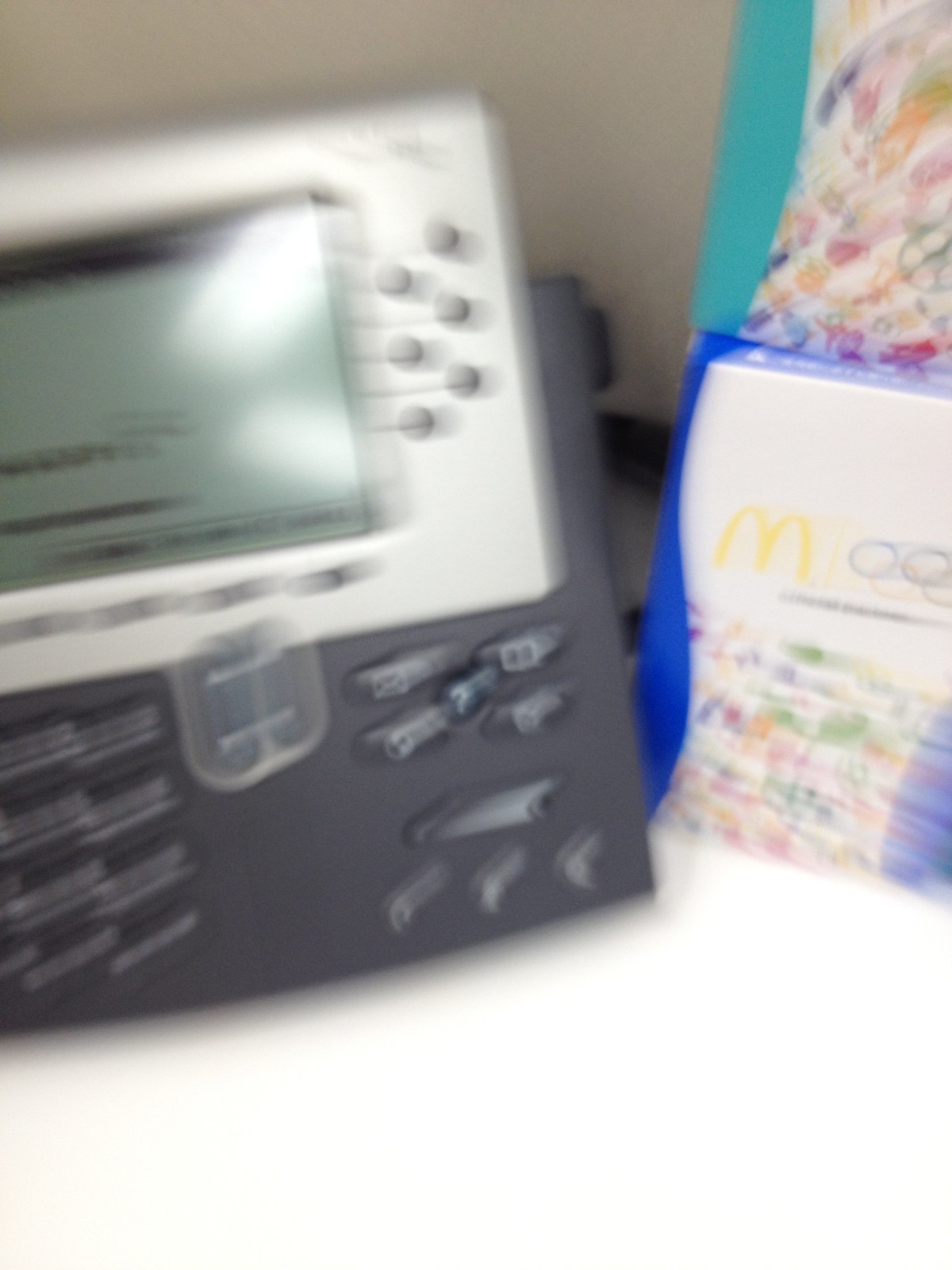This image showcases a somewhat blurry, angled view of a large gray box that appears to be a keypad or possibly an intercom system. The device has a prominent white section at the top, featuring numerous buttons, although the details are obscured due to the reflection of light on the surface. In the middle of the gray box, a clearer segment can be identified, appearing as a smaller box adorned with horizontal lines.

Adjacent to this main device, on the left side, is a McDonald's food carton. This carton prominently displays the Olympic rings among a variety of writing in multiple colors, including yellow, pink, and green, although the text is not discernable due to blurriness. On top of this McDonald's carton sits another carton with turquoise sides, which is also blurred, making it difficult to see specific details.